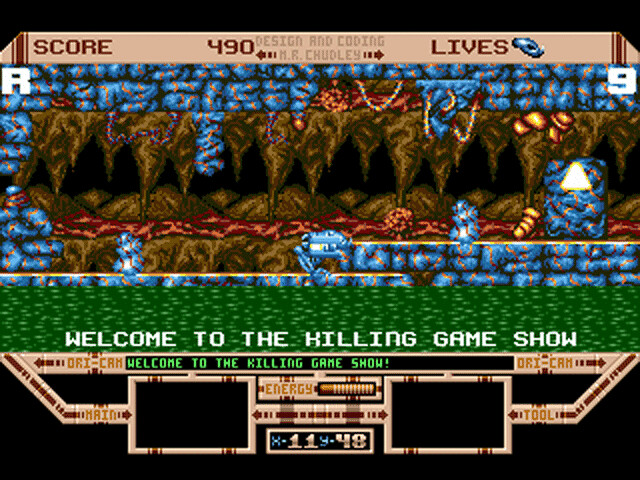This is a detailed screenshot of an 80s-era side-scrolling video game that takes place in an underground cave setting. The game interface is visually divided into several areas. 

At the top of the screen, there is a light brown banner displaying "SCORE" on the left with the value "490" to its right. Next to it, "Design and Coding Mr. Chudley" is written in gray, flanked by arrows, and a blue logo appears beside the word "Lives." The playing area of the game shows a dark, cave-like tunnel system, with brown and red rocky structures suggesting flowing lava, and blue stone adorned with yellow and orange lines. Stalactites hang from the cave ceiling, adding to the underground ambiance.

In the central part of the screen, amidst a green backdrop, bold text declares, "Welcome to the Killing Game Show" in both white and green letters, surrounded by tan and red interface elements. The lower section of the screen features elements of the user interface including energy levels and coordinates labeled as X11, Y48. Additionally, there are various UI components marked by an "R" in the upper left corner and "9" in the upper right, as well as a cryptic area displaying the words "Energy, dry cam, tool, main" just above coordinates indicating player position. The graphics are primitive, reminiscent of the 1980s gaming era, contributing to an overall nostalgic feel.